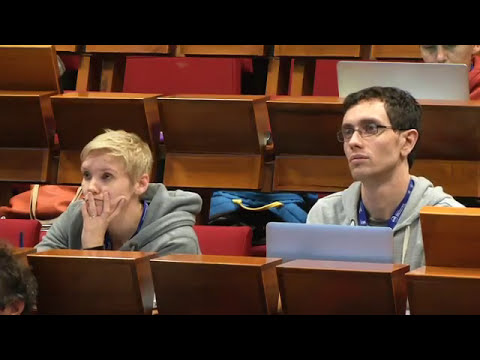The image, framed by medium-thick black borders at the top and bottom, depicts a classroom or college auditorium setting. In the second row, two individuals are seated, a woman to the left and a man to the right. The woman, with short blonde hair, wears a gray hoodie and has her left hand cupping her chin and covering part of her mouth and cheek. The man, sitting beside her, has short dark hair, glasses, and is dressed in a light jacket over a blue shirt. In front of him is an open laptop. On the floor behind them are two bags, one blue and one orange. In the upper right-hand corner, another open laptop partially obscures a person whose face is visible from the nose up, with the top of their head cut off at the border. The overall atmosphere suggests a learning environment, with brown, wooden-style desks and seemingly uncomfortable red seats.